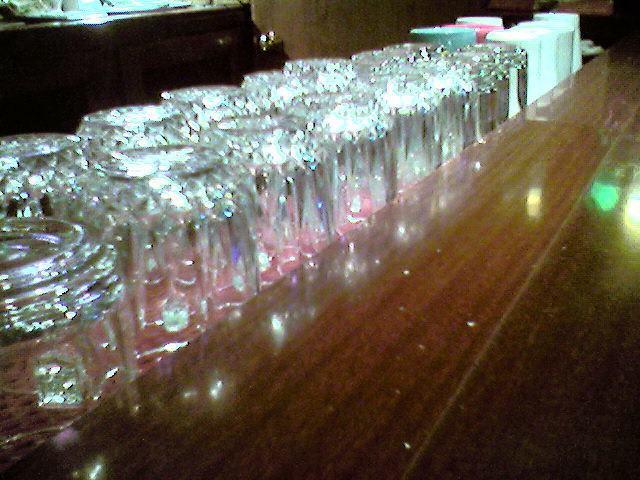The image captures an indoor setting of a bar, featuring a long, shiny wooden bar table. The table is neatly arranged with two rows of clean, upside-down glasses stretching from the left to almost the right side. Among these, there are several plastic cups in various colors: green, pink, and predominantly white. The polished wood reflects both the glasses and cups, creating light spots on its surface. Notably, there is a sequence of colored reflections: a yellow one, followed by a green one, and then a white one with a yellow hue around it. In the background, a cabinet can be seen with its upper part illuminated in shades of green, blue, and white. The entire photograph is rectangular, emphasizing the organized and reflective nature of the bar setting.